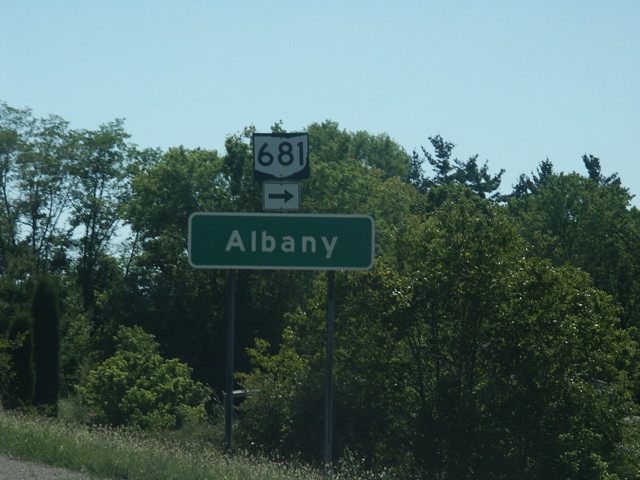The photograph, presented in landscape orientation, captures a somewhat overcast day with a clear view. The sky, a pale baby blue, stretches from the upper left to the upper right, providing a gentle backdrop. In the lower left corner, a patch of dirt transitions seamlessly into lush green grass, with outlines clearly visible and lightly tinged with shades of pale gray, yellow, and pink. 

Dominating the foreground, at the center-bottom of the image, stand two sturdy green poles that appear dark gray. These poles support a large, prominently displayed oval sign with rounded edges. The sign is green, bordered in white, and bears the inscription "Albany" in bold white letters. Above the sign, there is a dark black directional arrow pointing to the right, and above this arrow is the shape of the state of New York, indicating Routes 688 and 681 heading to the right. 

In the background, forming a natural frame from left to right, is a dense forest of trees, adding to the serene, rustic atmosphere of the scene.